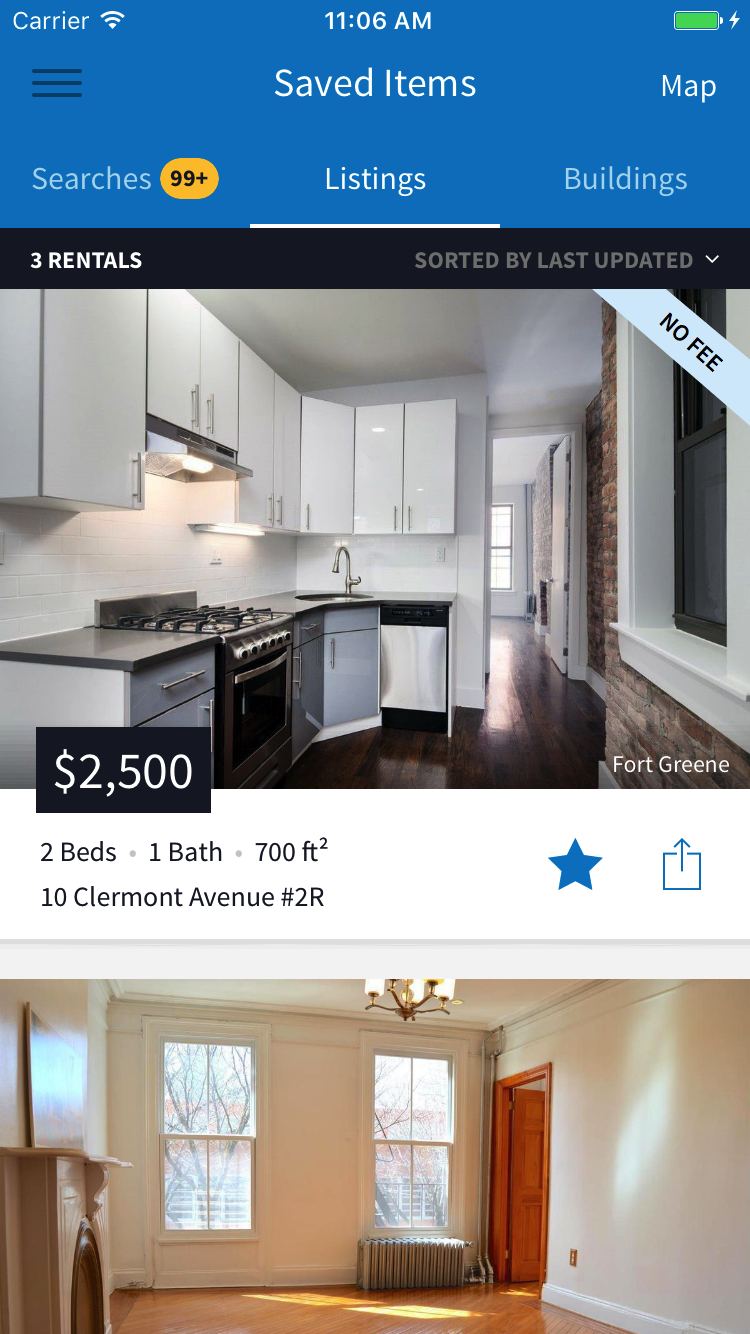"Vertical smartphone screenshot featuring a real estate app's interface. The top section displays a cerulean blue background with device status icons: 'carrier' with a Wi-Fi symbol on the upper left, the time '11:06 AM' centered, and a green battery icon with a white lightning bolt indicating charging on the upper right. Below this, a navigation bar features three horizontal black bars for additional options on the far left, followed by the text 'Saved Items' in white. On the same line, on the upper right below the battery icon, is the word 'MAP' in uppercase white letters.

To the left once again, the word 'Searches' is visible next to an orange circle with '99+' in black. The middle section highlights 'Listings,' which appears in bold with an underline, showing it as the selected tab. Adjacent to this is the word 'Buildings.' A black rectangular strip below these tabs contains 'Three Rentals' in white on the left side and 'sorted by last updated' on the right. 

The main content features a property listing with a photo of a kitchen. The listing details include a price of '$2,500,' specifying '2 beds, 1 bath, 700 sqft' and the address '10 Claremont Avenue.' Icons for 'star' to favorite and 'share' options are visible. Another smaller image showcases the living room, providing a comprehensive view of the property."